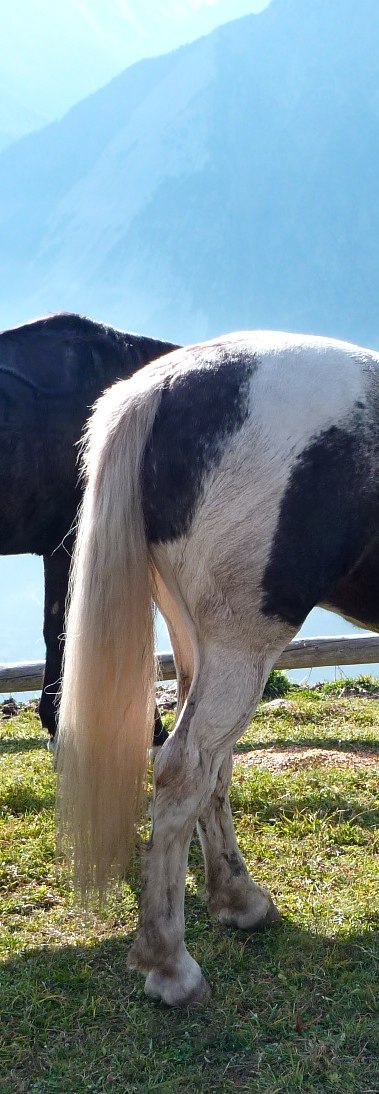The image captures a picturesque outdoor scene dominated by a majestic mountain in the distance, bathed in a hazy blue light. The mountain's rugged face features sections of dark rock interspersed with pristine white snow. In the foreground, the focal point is two partially visible horses standing on a lush, green cliffside. The brown and white horse with gray hooves takes the front, showcasing its long white tail. Positioned slightly behind is a black horse, also with gray hooves, partially obscured by the horse in front. The cliffside is detailed with green patches of grass and a wooden log that acts as a natural railing, its wooden grain clearly visible. Above, the bright blue sky is dotted with patches, providing a vibrant backdrop to this tranquil scene. Through the gaps between the horses and the log, glimpses of the sky enhance the overall composition.